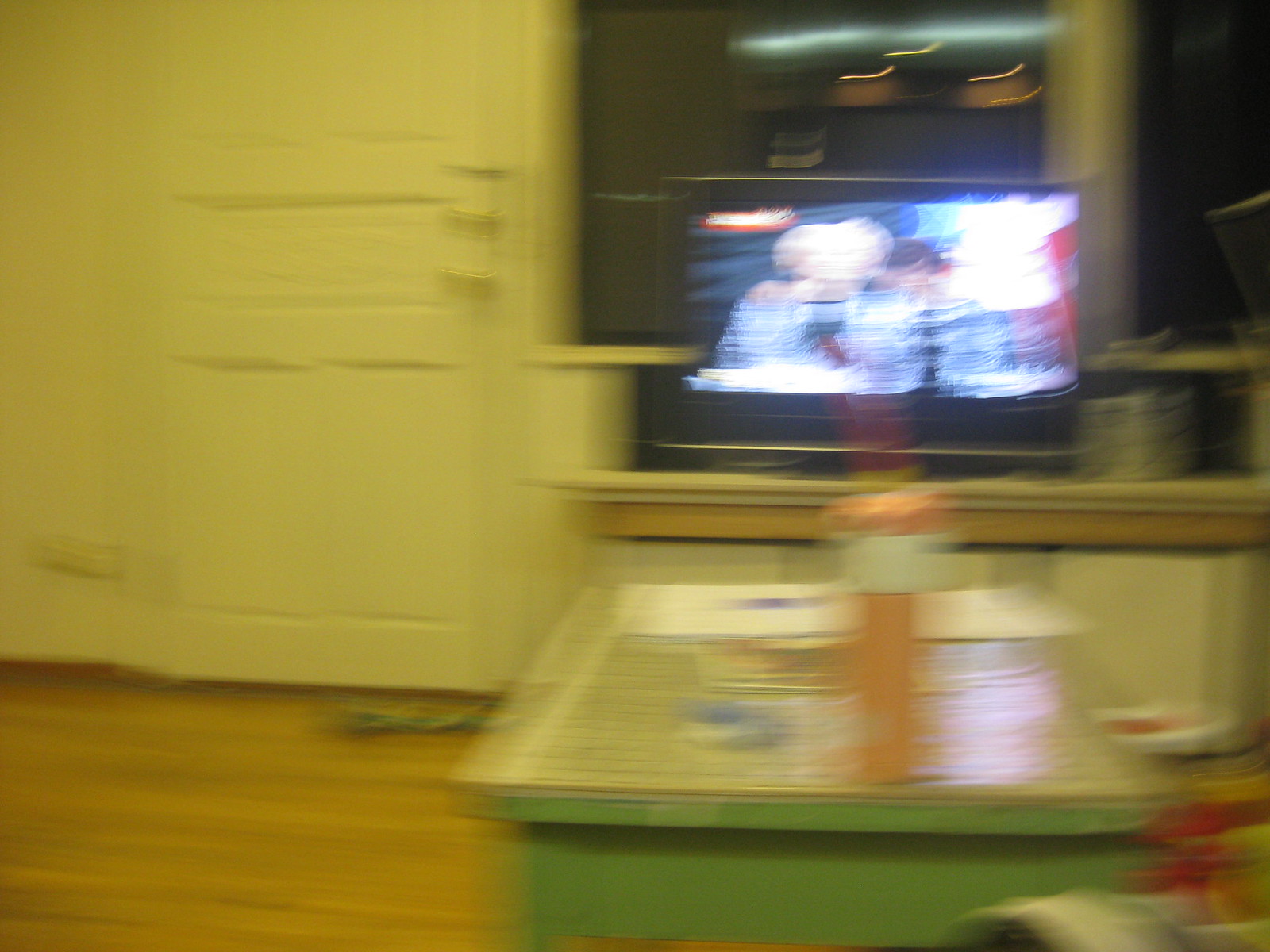A slightly blurred photograph of an interior room features light-colored wooden flooring. In the left background stands a white or perhaps cream-colored wooden door that appears yellowish. The foreground on the right showcases a green table or desk, adorned with an unidentified orange knickknack, a plate, and scattered papers with colorful markings. Behind the table, a TV is turned on, positioned on a wooden ledge. Beyond the TV, several windows can be seen, all revealing darkness outside.